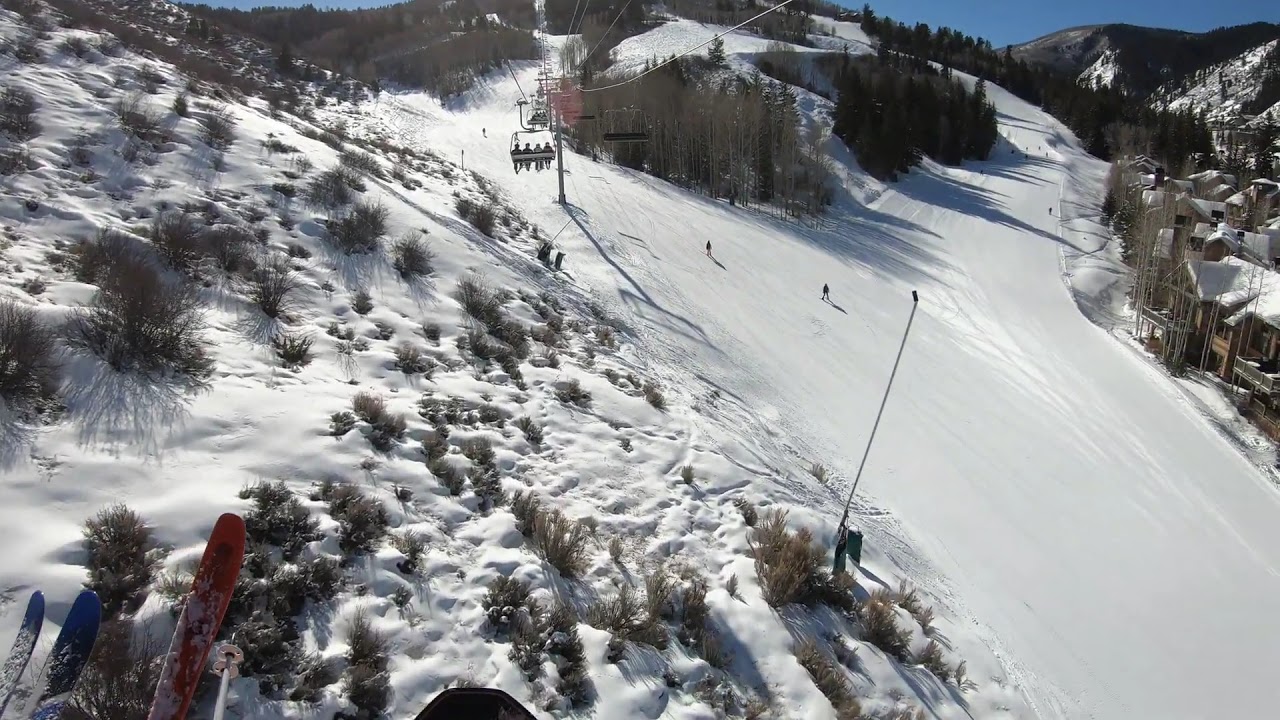A captivating photograph of a pristine ski slope captures a winter wonderland scene from an elevated vantage point. Dominating the center of the image, a ski lift runs diagonally with several benches occupied by skiers making their ascent. The left side of the picture features snow-covered terrain interspersed with rugged vegetation in shades of brown and green. On the right, the ski slope descends steeply, dotted with multiple skiers gliding down towards the bottom right corner. Flanking the slope's edges are two-story houses, their roofs blanketed in snow. The sky above is an unblemished light blue, providing a stark contrast to the distant mountain range, which shows barren, gray patches amid its own snowy cover. The bottom left corner of the photograph reveals the tips of two skis, one blue and the other red, with a mysterious silver pole extending from beside the red ski, adding an intriguing detail to the composition.